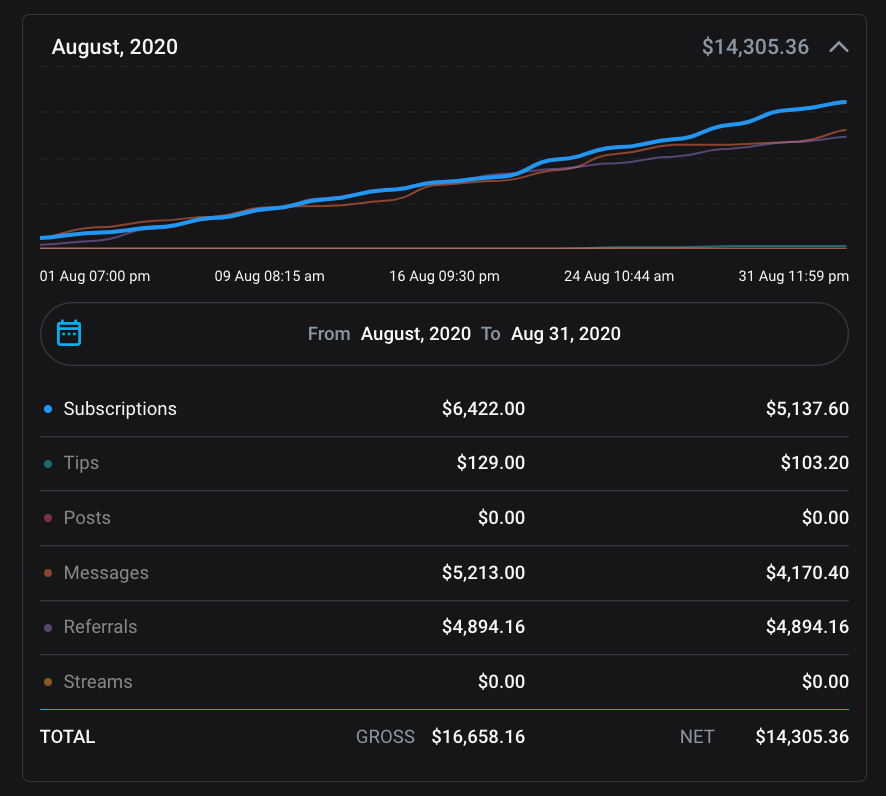The image features a black background and prominently displays the text "August 2020" along with a figure of "$14,305.36". Overlaying the background are three graph lines in blue, purple, and red, which correspond to different data sets. The x-axis is marked with specific timestamps: "1 August 7:00 p.m.", "9 August 8:15 a.m.", "16 August 9:30 p.m.", "24 August 10:44 a.m.", and "31 August 11:59 p.m."

Additionally, there is an oval that highlights the duration from "August 2020" to "August 31st, 2020". Below the graph, there is a detailed breakdown of various metrics for the month:
- Subscriptions: 6,422, generating $6,422.
- Tips: collected $5,137.60.
- Posts: 0, contributing $0.
- Messages: 5,213, totaling $4,170.40.

These values collectively amount to the displayed total of "$14,305.36" for the specified time period.